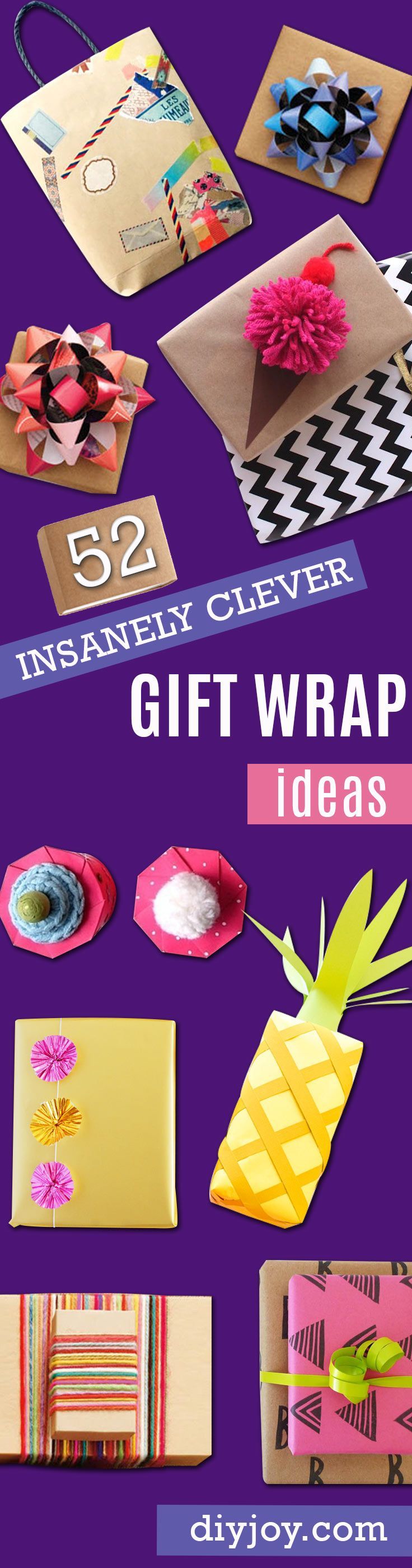The image is a tall, thin poster from DIYJoy.com with a dark purple background, prominently displaying the text, "52 Insanely Clever Gift Wrap Ideas." A multitude of smaller presents are showcased, each wrapped in unique and creative ways. Notable designs include a brown box with a blue bow, a box adorned with a pom pom and shaped to resemble an ice cream cone, a red box with crocheted items, and a rectangular package wrapped to imitate a pineapple. There's also a yellow box with pink and gold metallic decorations and a box entwined with numerous pieces of string. Some patterns are simple, such as brown paper gift wraps and boxes with bows, while others are less standout with semi-interesting designs. The image captures the essence of DIY gift-wrapping, encouraging creativity for those looking to make their presents visually appealing. The bottom of the poster is marked with "DIYJoy.com," signaling it as a gateway to a larger article on clever gift wrap ideas.